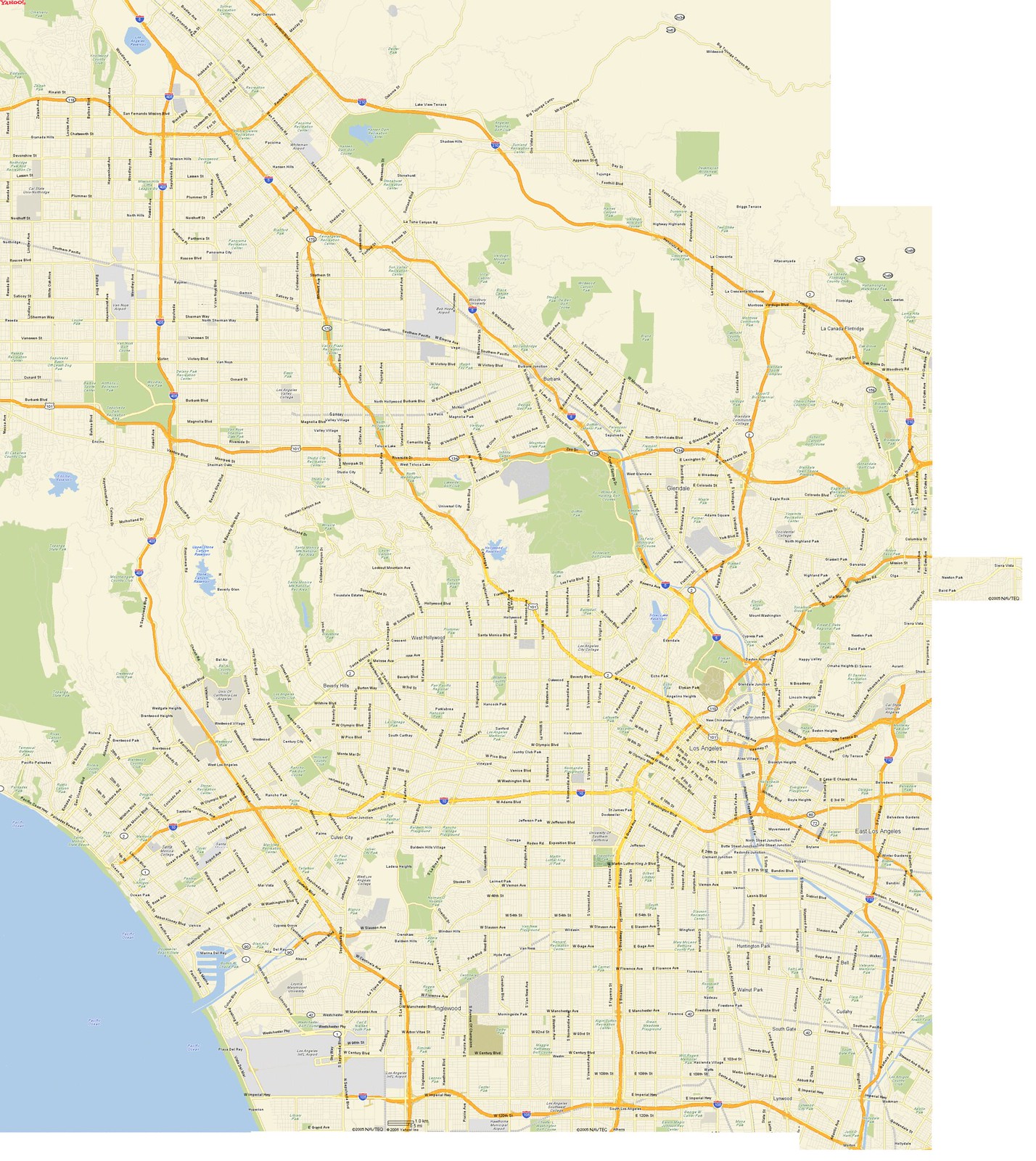This detailed map illustrates a metropolitan area with distinct geographical and infrastructural features. In the bottom right section, a body of blue water is prominently displayed. Moving towards the bottom, the landscape is crisscrossed with yellow lines representing roadways that traverse and meander through various structures and streets, typical of an urban grid.

Adjacent to the water on the bottom left, a gray zone is evident, likely denoting a built-up industrial or commercial area. Black annotations across the map provide street names and probable landmark locations, offering navigational aids and highlighting key areas within the city.

Scattered among the yellow-lined roads are bluish dots which likely indicate specific locations or points of interest, enriching the map with additional contextual information.

The top portion of the map lacks the yellow road markings seen below, instead displaying an off-white to greenish area, signifying less urbanized zones. These green patches are identified as forests and parks, with larger green spaces located at the top left and center, along with smaller scattered green areas. The bottom section of the map contains only one discernible green area, further emphasizing the predominantly urban nature of this region.